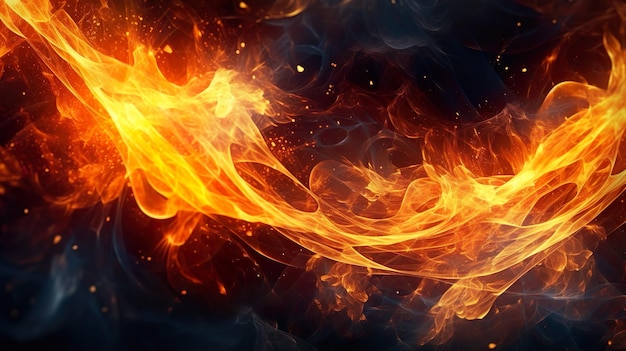The image is a horizontally rectangular digital artwork with no discernible border, set against a backdrop of deep darkness and swirling wisps of smoky hues. The primary visual element is a dynamic slash of fire that originates from both the upper left and right corners, converging toward the center about two-thirds of the way down. The flames showcase a vibrant palette of bright yellow, vivid orange, and deep orange-red tones, creating a highly animated and intense visual impact. The background consists of dark blue and dark orange clouds resembling stormy plumes, interspersed with sporadic pinpoints that appear to be sparks. The smokey backdrop features pillaring and swirling gray and black wisps that enhance the fiery spectacle in the foreground. The interplay of light and dark, coupled with the intricate details of fire and smoke, gives the impression of a powerful, almost otherworldly conflagration. No text or artist's signature is present to provide additional context.